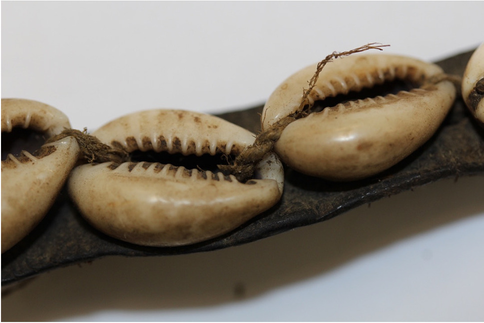In this detailed close-up image with a gray background, we see a rectangular photograph featuring a piece of craftwork that closely resembles a bracelet or possibly another form of jewelry such as an anklet or necklace. Dominating the composition is a brown leather strap, which extends diagonally from the lower left corner to the upper right. Atop this leather band are three to four small, round, cream-colored shells with darker brown edging around slit openings. These openings reveal a brown cord or twine that intricately weaves in and out, securing the shells to the leather strap. Each of the shells is identical, smooth, and sits in a linear arrangement, linked together by the twine. Shadowing beneath the leather band adds depth to the image, accentuating the texture and craftsmanship of the piece. The overall impression is one of a delicately handcrafted item, possibly a homemade accessory, artfully displayed against its neutral backdrop.